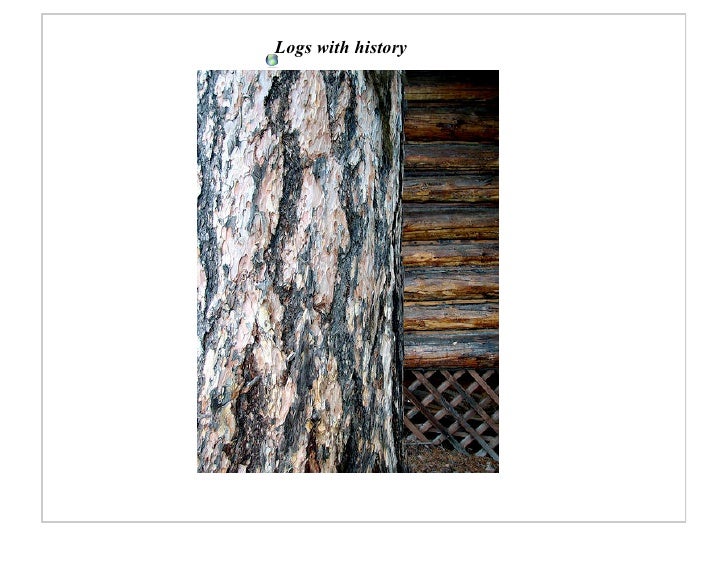This image features a detailed view of a vertically oriented tree log occupying the left half of the frame, showcasing a natural bark texture with shades of brown, gray, black, and a hint of green. The bark has scaled, cracked patterns, enhancing its rugged appearance. In the right portion of the image, we see a log home constructed with round logs running horizontally. These logs are darker brown, possibly coated with some veneer or sealant, and interspersed with what appears to be black tar or pitch. Below these horizontal logs, there's a painted brown lattice, adding depth and contrast to the image. The background remains predominantly white, emphasizing the subjects. At the top of the image, in black letters, is the caption "logs with history," suggesting a narrative element to the objects depicted.